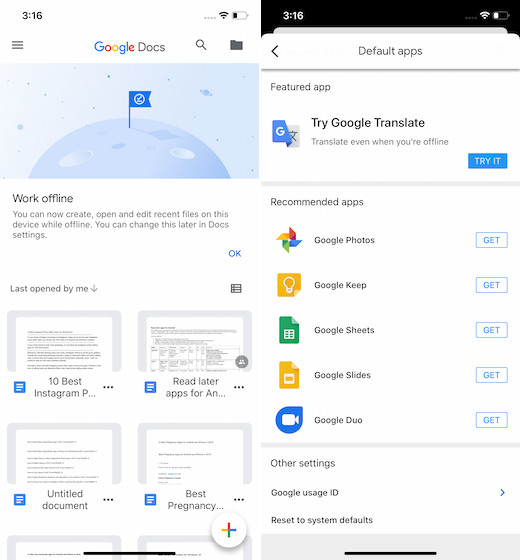This is a screen capture featuring two side-by-side images of different Google apps on an iPhone, showcasing their interfaces and functionalities. 

On the left side, the app displayed is Google Docs. The top ribbon features the usual icons for functions such as battery status, Wi-Fi, and time. The main focus of the screen shows the Google Docs logo with a banner image of "Cartoon Planet" accompanied by a blue flag icon. Below this, there is a highlighted message stating, "Work offline - You can now create, open, and edit recent files on this device while offline. You can change this later in Docs settings." Beneath this message, the interface displays two columns of various documents under the heading "Last opened by me." The first document listed is titled "10 Best Instagram." Below it, there is an "Untitled Document." To the right, additional documents are listed with titles such as "Read Later Apps for..." and "Best Pregnancy."

On the right side, the app displayed is the Google Play Store, focusing on Google Translate. At the top, there is a featured app section with the message, "Try Google Translate - Translate everything when you're offline." There is a prominent blue button labeled "Try it" in the lower right of this section. Below this are recommended Google apps, including Google Photos, Google Keep, Google Sheets, Google Slides, and Google Duo, each followed by a "Get" link for easy download.

Together, these images illustrate the layout and key functionalities of Google Docs and the Google Translate promotion within the Google Play Store, highlighting the offline capabilities and various Google apps available for download.